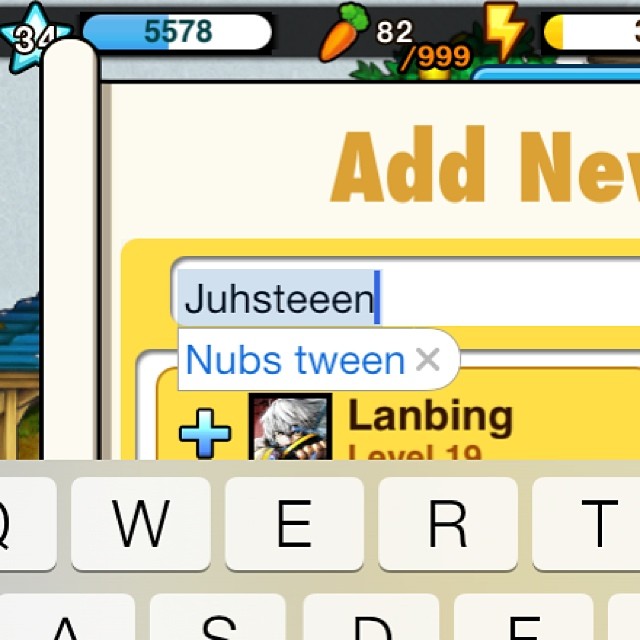The image depicts a close-up screenshot from a mobile game displayed on a device, with the lower part of the screen showing portions of a beige Mac keyboard, specifically the keys QWERT and the top of ASDE. At the top left of the screen, there's a significant detail featuring the number 34 within a blue star, which appears to display the player's level or a similar status. Adjacent to it is a progress bar showing 5778, possibly indicating points or progress in the game, with the bar partially filled in blue. Next to this, there is a cartoon icon of a carrot accompanied by the numbers 82/999, suggesting the player has 82 out of a possible 999 carrots collected. Further to the right is a small yellow lightning bolt with an almost empty progress bar underneath, indicating some form of energy or power level. Below these details, there is a search bar with the letters J-U-H-S-T-E-E-E-N typed in, which auto-corrects to NUBSTWEEN. Adjacent to the search bar, an avatar icon is visible, flanked on the left by a blue crossmark and on the right by the words "Lanbing, level 19." The visual elements suggest a game interface with various progress indicators and interactive elements.